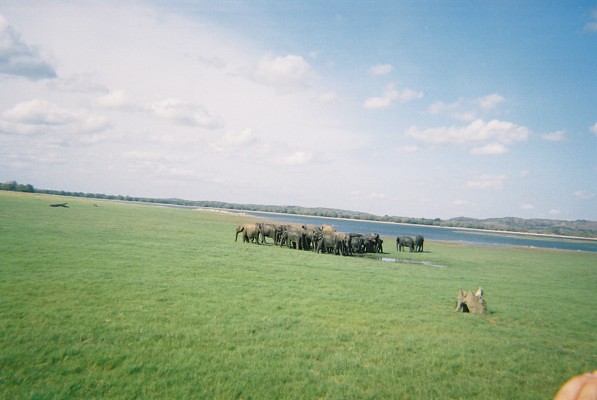The image captures a vibrant outdoor scene with a sweeping view of nature. The upper half of the image is dominated by a dynamic sky, transitioning from a darker blue on the right to a lighter blue on the left, filled with fluffy white clouds that are more concentrated on the left side. In the distance, a strip of land, adorned with trees and a hill, lies beyond a serene body of water. Moving towards the foreground, there is a vast, lush green field teeming with wildlife. Though the animals are small, they appear to be a herd of about 20 to 25 elephants, identifiable by what look like trunks hanging down. The scene also includes some indistinguishable light brown or tan animals. Notably, in the very bottom right corner, a portion of the photographer’s thumb is visible, hinting at the candid nature of the shot.